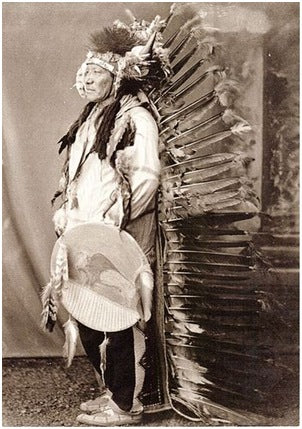This sepia-toned photograph features a Native American man in a nearly profile view, facing left. He is adorned in traditional attire, highlighting a long feathered headdress, or war bonnet, that cascades down to the floor. His hair is intricately braided over his shoulders, and he wears a large white shirt. The man holds a flat, drum-like round object made of buckskin, adorned with feathers along its edges and featuring a small illustration of a buffalo. The background suggests he is outdoors, as indicated by the visible dirt and rocks, and he appears to be seated or standing next to a tent. The backdrop is a plain cloth, emphasizing his neutral, stoic expression and traditional regalia.